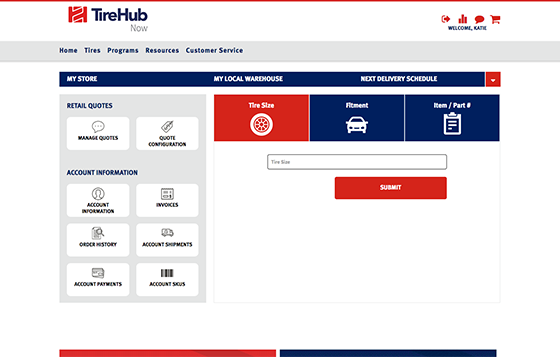The image showcases the homepage of the Tire Hub website. Prominently displayed in the top left corner is the company's name, "Tire Hub." To the right, in the top right corner, are three navigational buttons labeled "Tire Size," "Alignment," and "Item and Part." Beneath these options is a search bar accompanied by a Submit button. On the left side of the page, there's a vertical menu offering additional navigation options, including links for Account Information, Invoices, Order History, Account Statements, Account Payments, and Account Services. The bottom right corner features a large open space, likely intended for main content display. The webpage has a clean white background accented with blue and red buttons. Beneath the company's name in the top left, there are five links to various sections of the website: Home, Tires, Programs, Resources, and Customer Service.